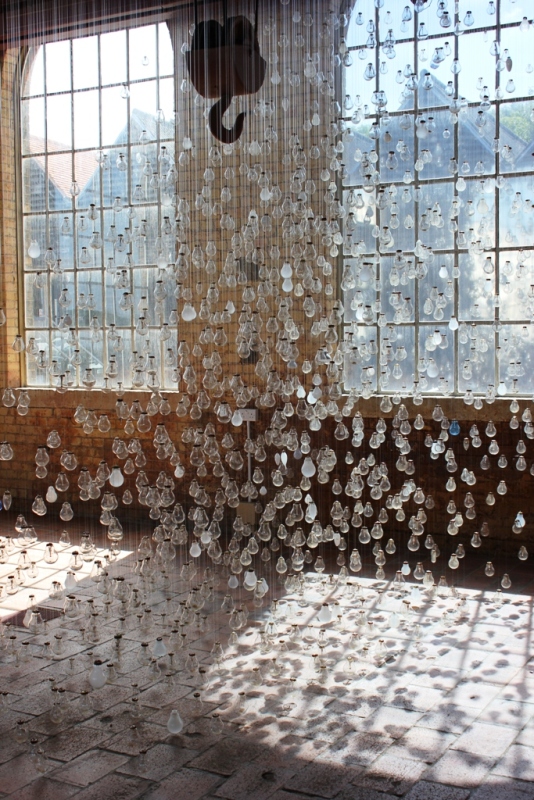The image features an interior scene with two large, multi-paned windows framed by wooden structures. Between the windows hangs a prominent, large black hook from the ceiling. This hook is reminiscent of those used in meat houses or for hanging heavy bags of hay, but it currently holds nothing. The background includes a cement brick floor and a brown wall separating the windows. Covering the entire scene from top to bottom, side to side, are countless tear-shaped beads suspended from the ceiling on threads, creating the illusion of falling raindrops. These beads condense more densely towards the bottom, forming an almost opaque barrier. Despite this, you can faintly see two large houses outside the windows, indicating life beyond this somewhat surreal, indoor raindrop-like phenomenon.